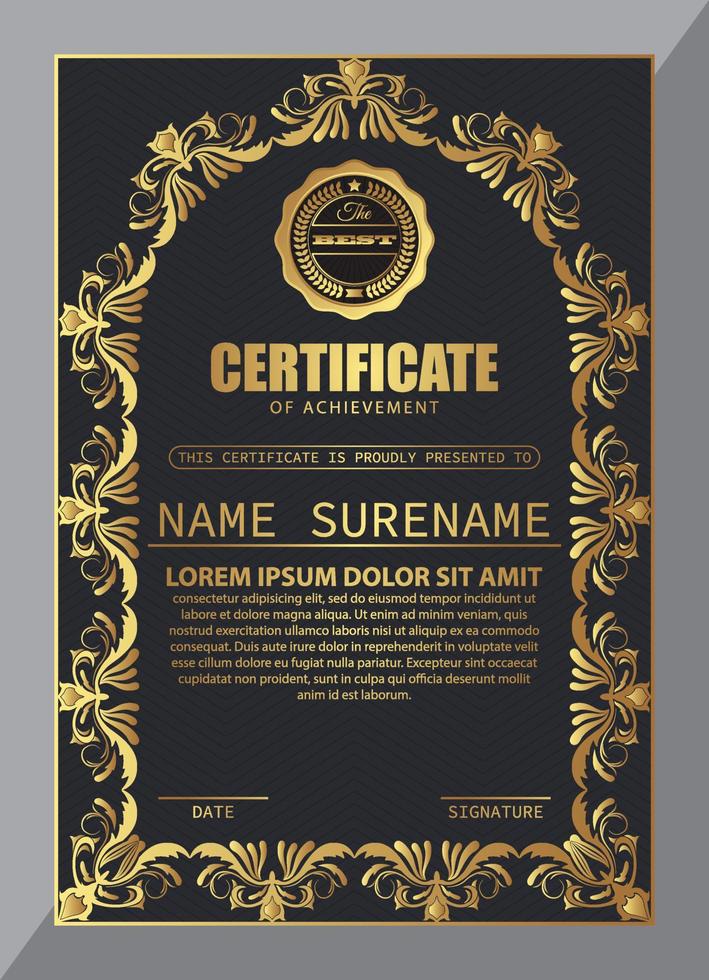The image showcases a highly polished mock-up of a certificate, likely intended to symbolize a diploma or an award. It features a striking design with a predominant black background accented by various hues of gold, ranging from lighter to darker shades. Framing the certificate is a thin, elegant gold border, further encircled by a subtle gray border, giving an impression of depth and sophistication.

At the top of the certificate is a circular crest adorned with olive branches and topped by a star, within which the word "Best" is prominently displayed. Below the crest, in bold and professional gold text, it reads "Certificate of Achievement," followed by a statement "This certificate is proudly presented to." There's a placeholder for a recipient's name displayed as "Name Surname," followed by a line meant for the actual name entry.

Further down, the layout includes a paragraph of placeholder text in Latin ("Lorem Ipsum Dolor Sit Amet"), which is in gold and slightly faded, indicating a space for supplementary information or commendations. Below this text are two distinct gold lines: to the left, a line for the date, and to the right, a line for a signature. The entire design is meticulously cropped and shows linear patterns throughout, emphasizing its modern yet professional feel. The certificate's intricate details and layered borders suggest it could be easily digitized and printed, making it both a visually appealing and practical design.